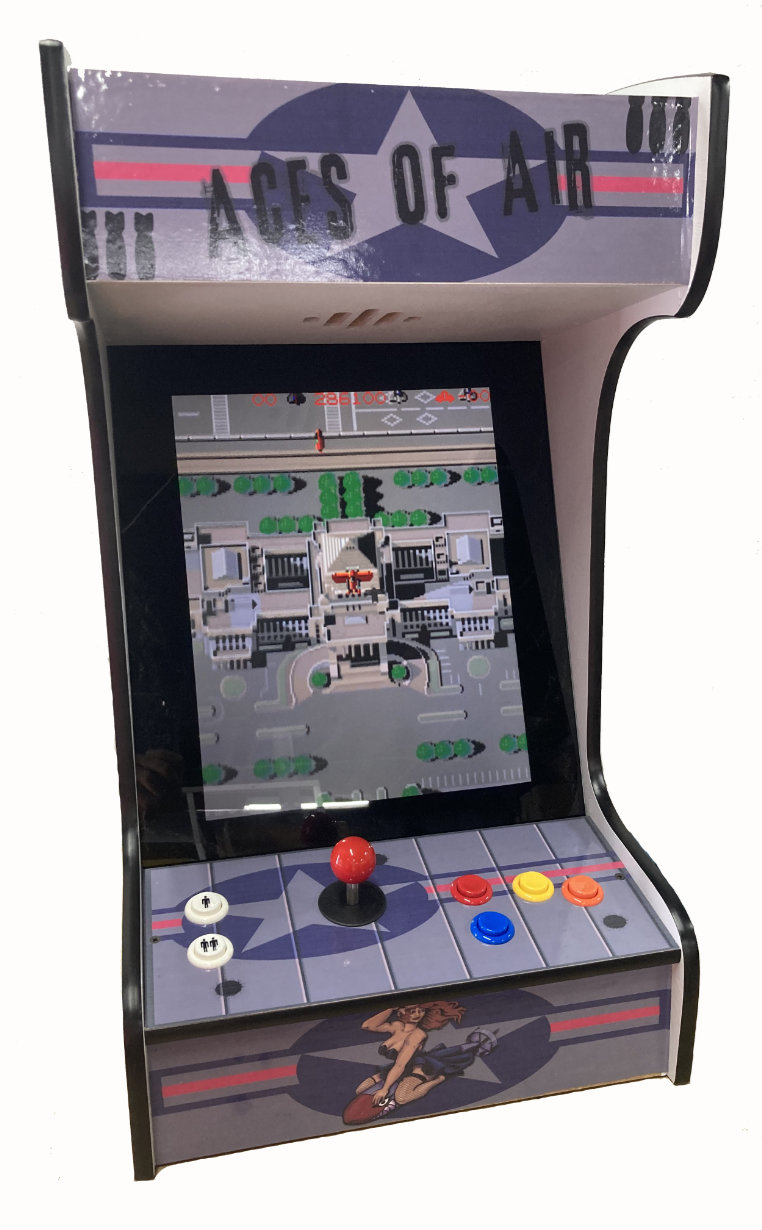The image depicts an old arcade cabinet for the video game "Ages of Air," prominently featuring a military theme. The marquee at the very top displays "Ages of Air" against a gray background, accented by a blue circle, a military star, and a pink stripe. Flanking the title are small bomb icons, three at the top and three at the bottom, with the title "Ages of Air" written in bold black text. The game screen showcases an overhead view of a terrain with roads, greenery, and gray structures. 

The control panel below the screen includes a red joystick flanked by player indicators: white stenciled icons for one and two players. To the right of the joystick, there are four colorful buttons - red, blue, yellow, and orange - set against the same background as the top panel. At the very bottom of the cabinet, there is an illustration of a scantily clad woman on her knees with flowing hair, touching her hair with one hand and resting the other on a brown object, adding an anachronistic element to the otherwise military-oriented theme.